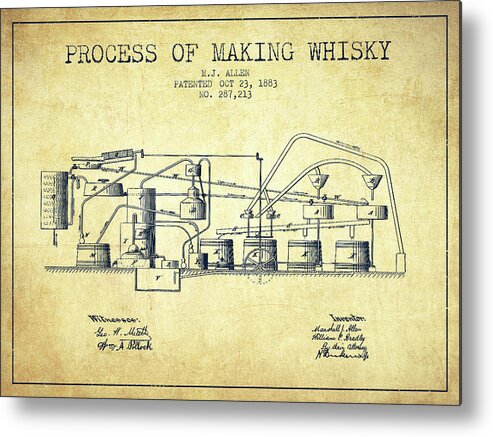The image depicts a detailed, black-and-white, typewriter-font diagram titled "Process of Making Whiskey" in all caps at the top. Below this title, in a smaller font, it reads "MJ Allen, patented October 23rd, 1883, number 287,213." The diagram intricately illustrates the whiskey production process, showcasing various cylindrical and cone-shaped mechanical components that resemble an assembly line. The background of the image is designed to appear as aged, yellowed, and speckled paper with brown splotches, adding to its antique look. A thin black line borders the edges. At the bottom, there are several signatures scattered on the left and right sides, adding to the document's historical feel.